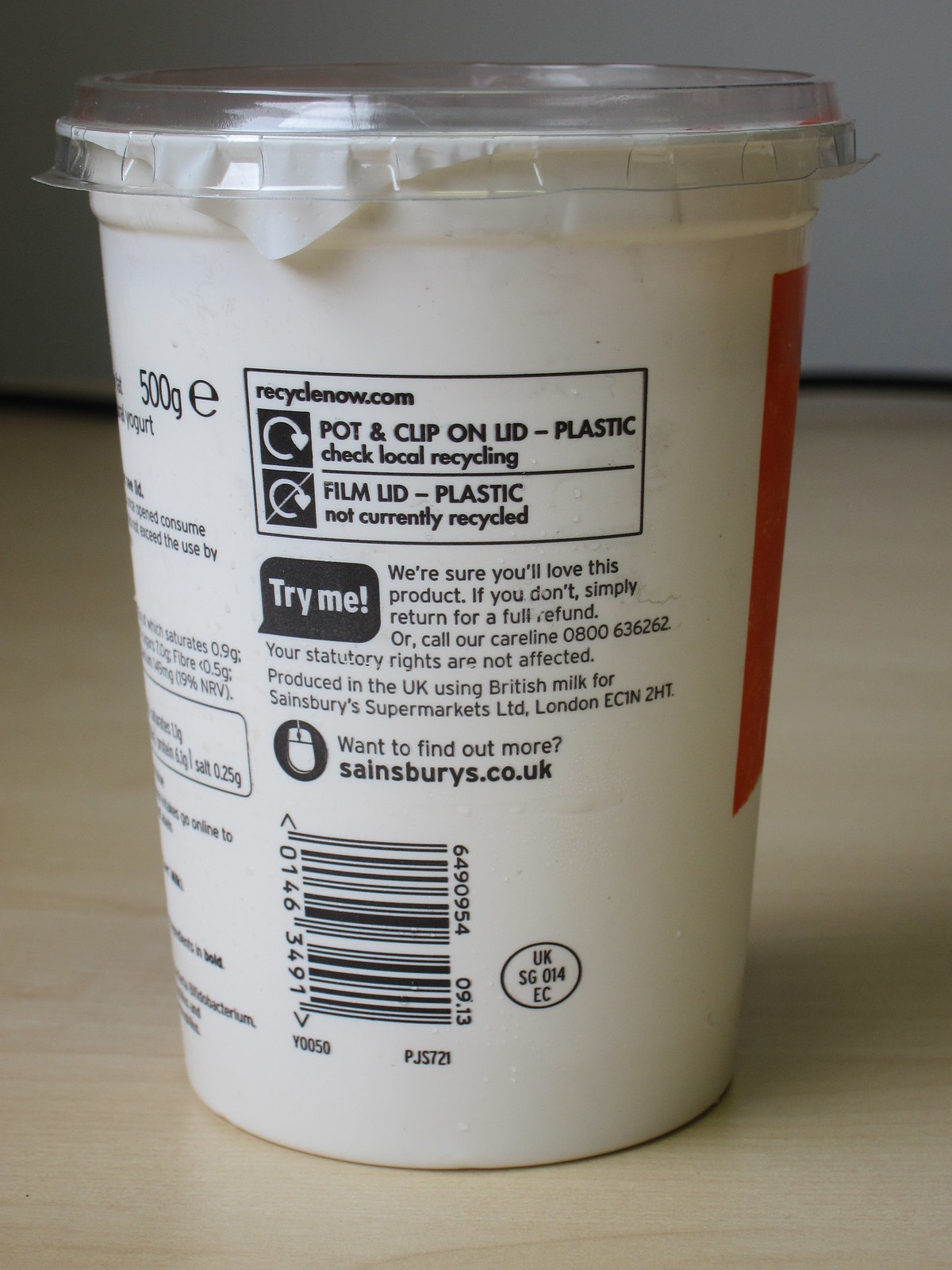The image showcases a white, cylindrical container, likely a tub of yogurt or a similar dairy product, with a clear plastic lid sealing the top. The container, placed against a cream-colored surface with a white wall in the background, features detailed labeling on its side. Prominently displayed is a box containing the web address RecycleNow.com, with icons indicating recycling information; the first icon notes "Pot and clip on lid: Plastic. Check local recycling," while the second states "Film lid: Plastic. Not currently recycled." Below these, a black speech bubble exclaims "Try me!" in white letters, accompanied by the reassurance, "We're sure you'll love this product. If you don't, simply return for a full refund. Or call our care line 0800-636-262. Your statutory rights are not affected." The label also specifies that the product is "Produced in the UK using British milk for Sainsbury's Supermarkets Ltd, London EC1N 2HT." An invitation to discover more information is provided with the URL Sainsburys.co.uk, situated above a UPC barcode positioned towards the center-left area of the container.